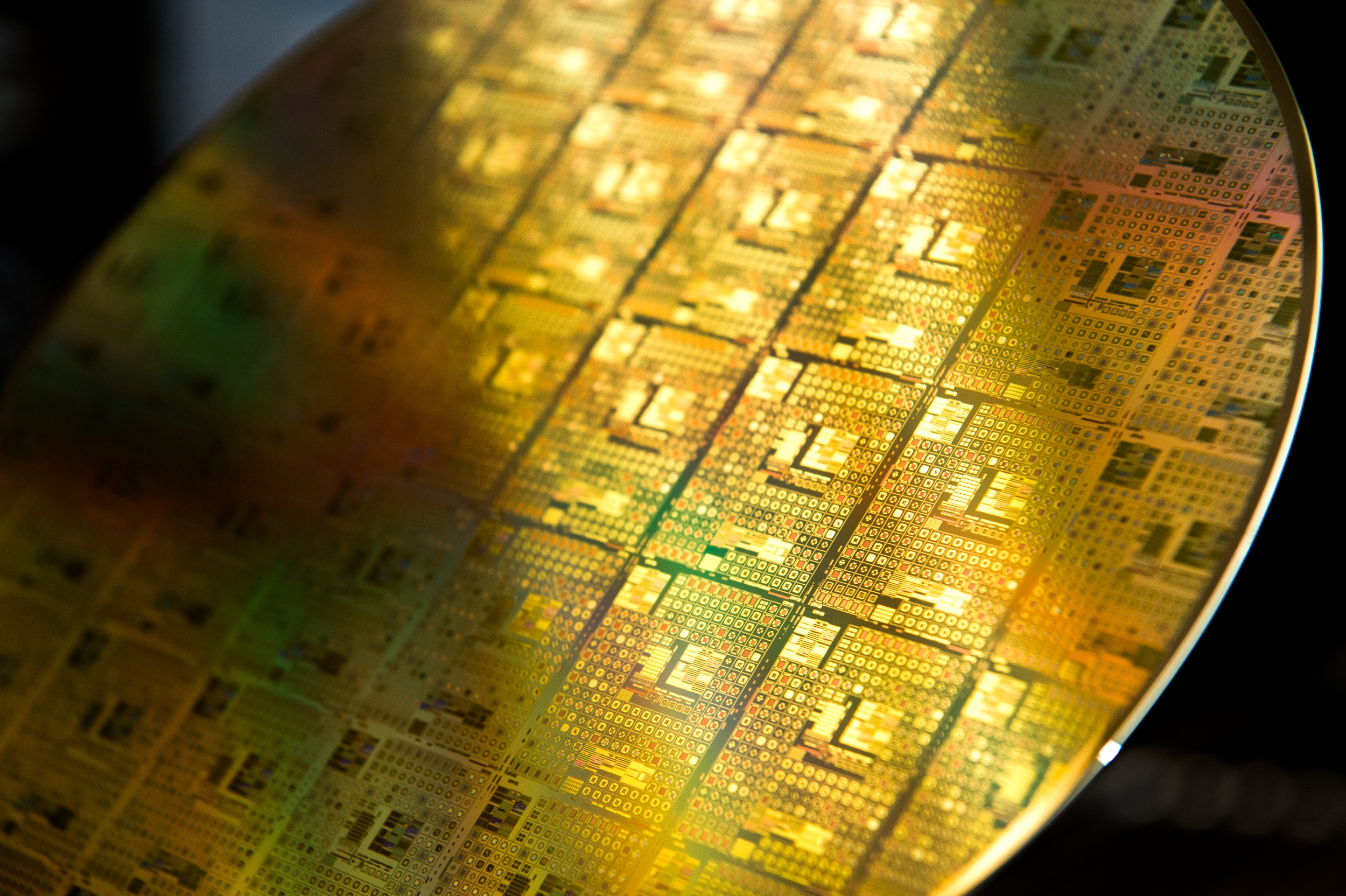This close-up photograph captures a circular structure that strongly resembles a gold disc with a grid-like pattern, evoking the intricate design of a microchip or printed circuit board. The circular object, which is thin and coin-like in shape, features a network of flat, square, and rectangular components in various colors, such as orange, black, and white, some of which are interconnected with tiny, precise circuitry. These elements are arranged in a clear five-by-five grid, creating a meticulous layout of larger and smaller squares within the overall circular form. The disc is bathed in light that primarily highlights its center, leaving the top left portion in shadow. Enclosed by a circular metal border, the disc sits against a dark background devoid of any text or additional imagery, emphasizing the detailed and complex nature of the components and circuitry within.